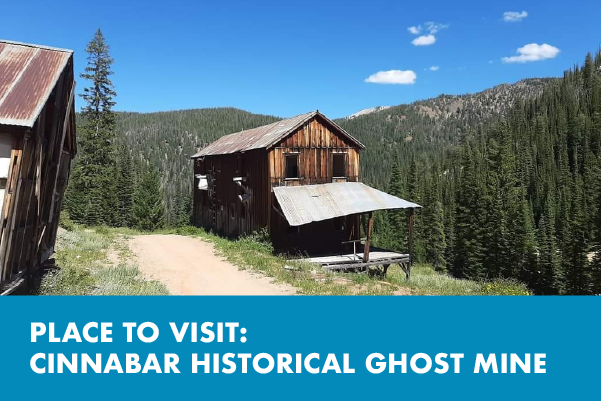The image resembles a postcard depicting the Cenobar Historical Ghost Mine, a notable landmark featuring two derelict wooden buildings. Both buildings are brown, constructed from weathered wooden panels, and stand amidst a dense grove of green evergreen pine trees. The larger building, perched at the edge of a hill with a mountain backdrop, is two stories tall, while the smaller, single-story cabin sits to its right. A pathway runs between the two structures, adding to the scene's rustic charm. At the bottom of the image, a teal blue rectangle houses white, all-capitalized text reading "PLACE TO VISIT CENOBAR HISTORICAL GHOST MINE."